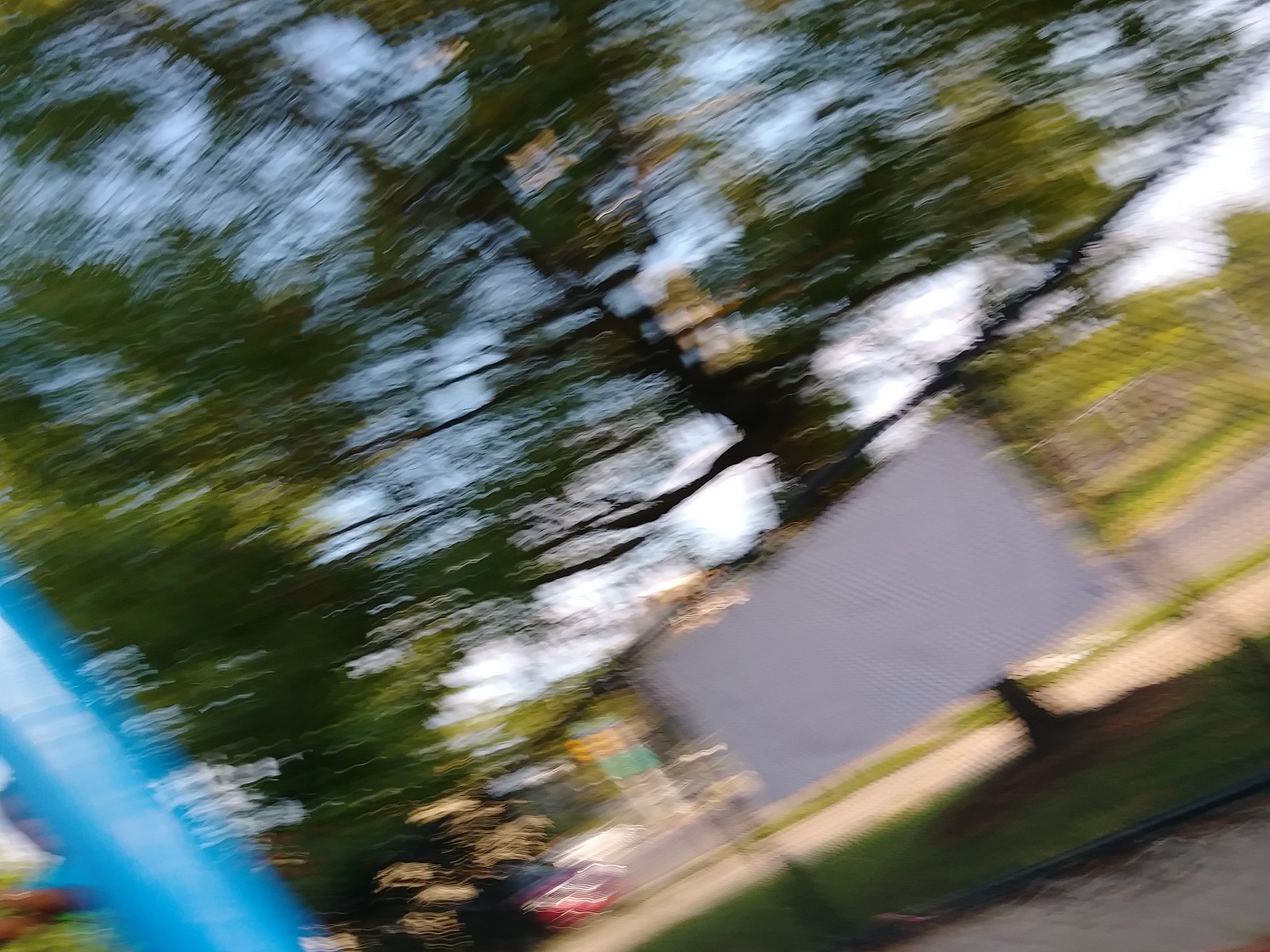A blurry outdoor scene featuring a lush green tree with blue sky peeking through its leaves occupies the upper left quadrant and central part of this image. A black, net-like substance overlays the tree. Toward the bottom right of the photograph, there's a white billboard propped up by two sticks, with the tree's trunk visible behind it. In the background, a commercial lot, possibly a shopping center, is visible. This lot features a red car and various store signs. A thick, neon blue line runs across the bottom left corner of the image.